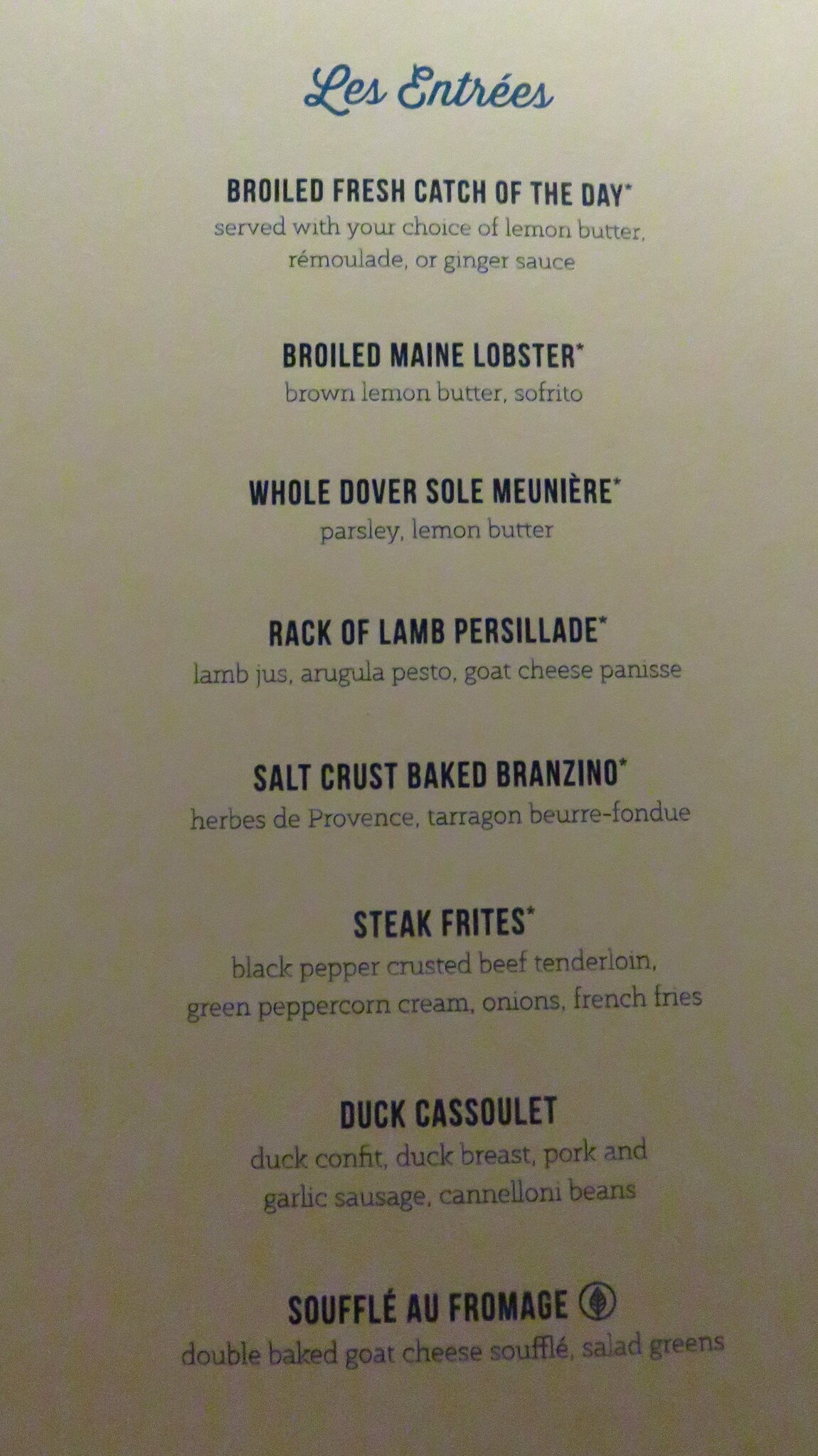This is an image of a portrait-oriented menu set against an off-white background that transitions from brighter at the top to slightly darker at the bottom. Centered at the top in yellow cursive text, it reads "Les Entrées." Below this heading, the entrées are listed in black text, each separated by some space. The first entrée is "Broiled Fresh Catch of the Day," served with your choice of lemon butter, remoulade, or ginger sauce. Next is "Broiled Maine Lobster," accompanied by brown lemon butter and sofrito. Following this is "Whole Dover Sole Meunière," paired with parsley lemon butter. The fourth option is "Rack of Lamb Persillade," featuring lamb jus, arugula pesto, and goat cheese panisse. Then there's "Salt Crust Baked Branzino," prepared with herbs de Provence, tarragon, and beurre fondue. "Steak Frites," plated with black pepper-crusted beef tenderloin, green peppercorn cream, onions, and french fries, is marked with a little star. The penultimate entrée is "Duck Cassoulet," which includes duck confit, duck breast, pork and garlic sausage, and cannellini beans. Lastly, there is "Soufflé au Fromage," a double-baked goat cheese soufflé served with salad greens, indicated by a leaf icon signifying it as a vegetarian option.